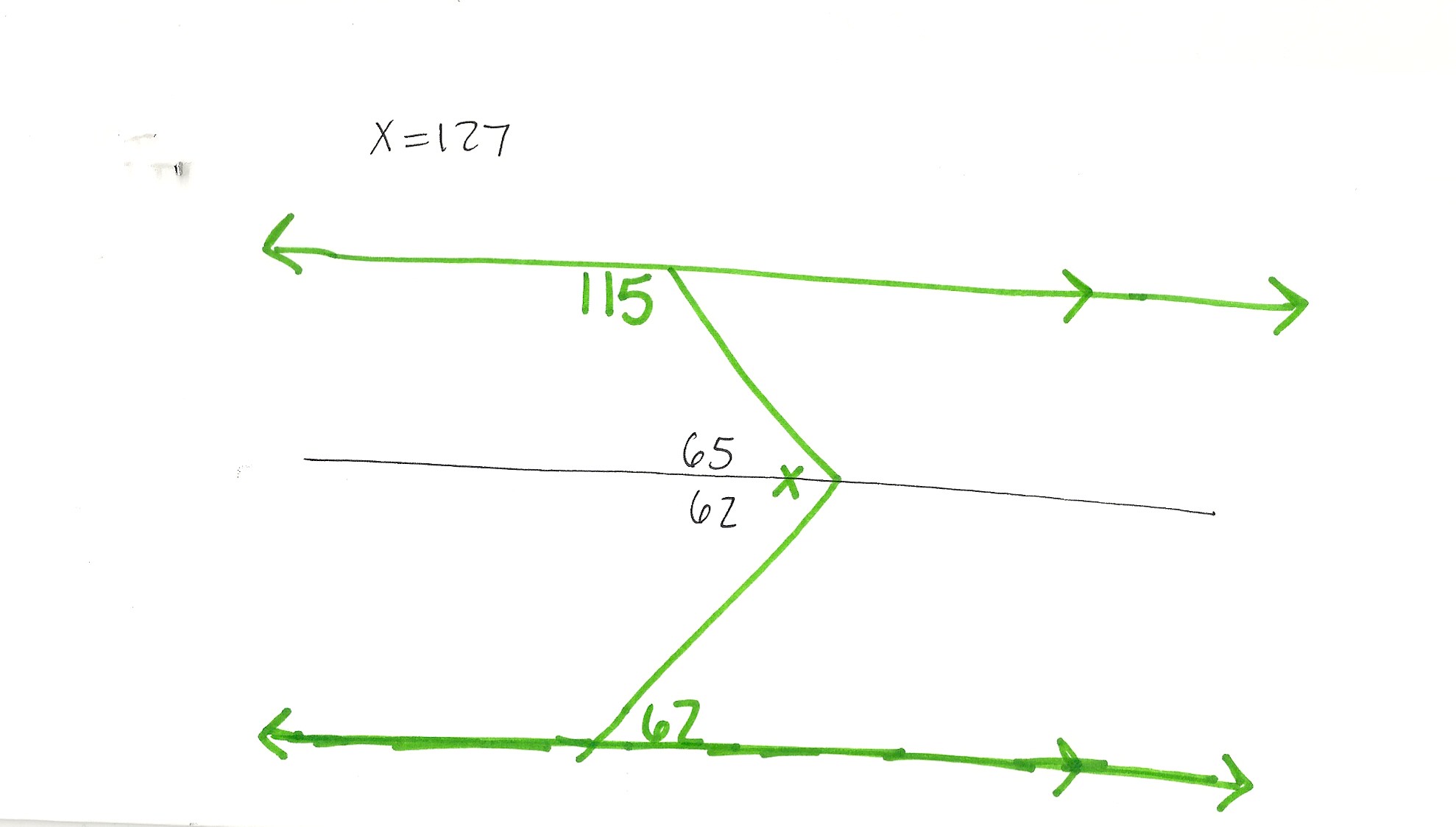A detailed diagram is presented on a white background. In the upper left corner, the text "X = 127" is written in black marker. Below this, an arrow drawn in green points to the left, connected to a horizontal line stretching across the image to the right side, where it terminates in a right-pointing arrow. Approximately two inches from this right-pointing arrow, another right-pointing arrow is indicated.

Near the middle of the image, towards the left side, the number "115" is written in green. It connects to a diagonal line slanting down and to the right, intersecting with a black horizontal line that extends from the left to the right side of the image. Along this black horizontal line, a green "X" marks the point of intersection. Positioned above the horizontal black line is the number "65" in black, while the number "62" in black appears below it.

Another green diagonal line originates from the first diagonal line's intersection and descends to the bottom of the image, intersecting with a bottom horizontal line. This lower horizontal line features green arrows at both ends, indicating leftward and rightward directions. The number "62" is written in green on the diagonal line at the intersection with the horizontal line. The bottom horizontal line also extends to the right, culminating in another right-pointing arrow, with an additional right-pointing arrow situated about two inches before reaching it.